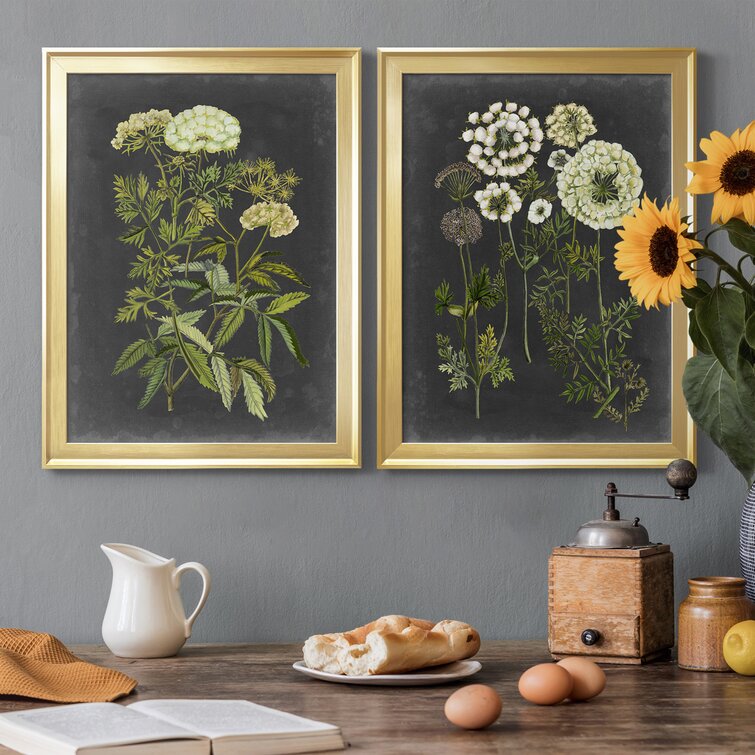This captivating photo, reminiscent of a home decorating magazine or a chic farmhouse cookbook, features a beautifully styled rustic scene. Two intricately framed floral paintings adorn a gray wall; both frames are gold-brown, enhancing the delicate artistry. The left painting showcases cream-colored tufted flowers with detailed leaf patterns resembling ferns against a green backdrop. The right painting features similar floral artwork, with elegant white flowers and intricate leaves set against a dark green background.

Beneath these paintings, a mixed wood table—a blend of dark and light hues—holds an array of charming, farmhouse-inspired items. At the center is a white plate holding a piece of homemade bread, surrounded by three farm-fresh brown eggs and a brown napkin. Adding to the rustic appeal, an antique, hand-cranked coffee grinder stands near a small jar, likely filled with coffee.

Completing the tableau are several elements that heighten its cozy farmhouse vibe: an open book, a cream-colored carafe, and a vase of realistic-looking sunflowers with deep green leaves grace the right side of the table. The overall aesthetic is a perfect blend of simplicity and elegance, reminiscent of a classic yet classy farmhouse scene.